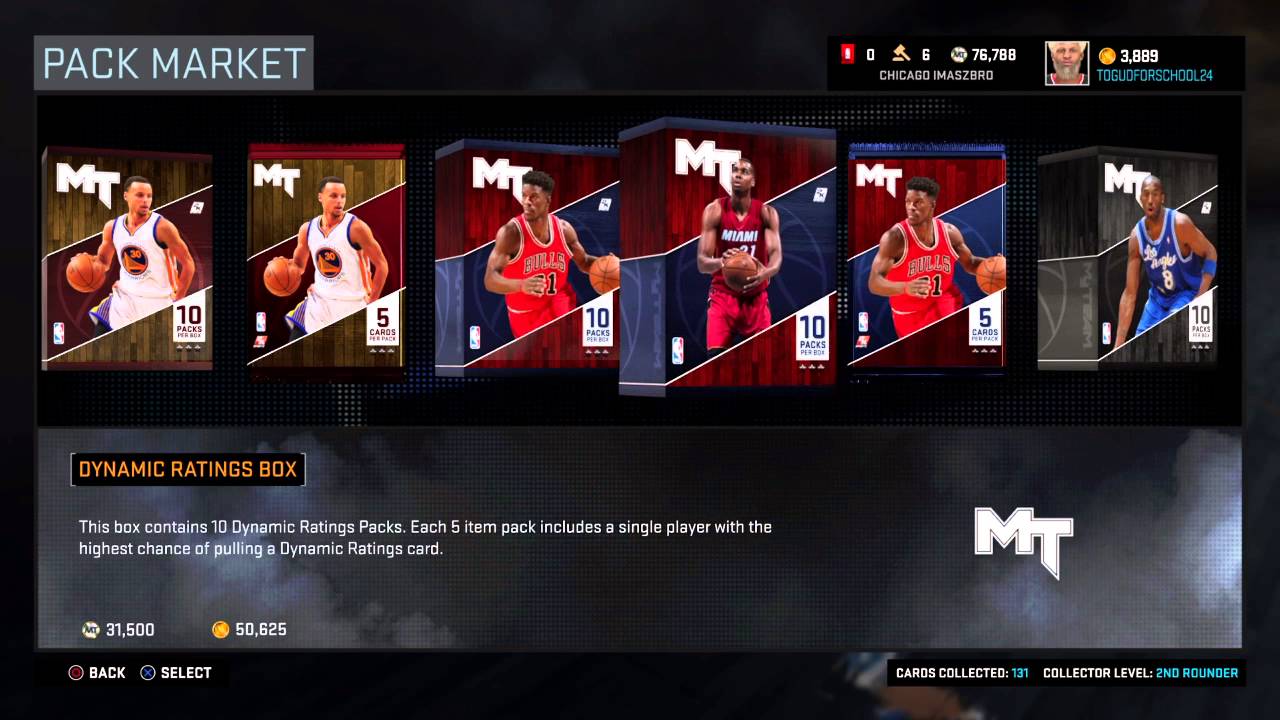This is a detailed screenshot of a PlayStation basketball video game interface, identifying key elements and functionalities. The lower-left corner displays two button prompts: the 'back' option with the PlayStation circle button and the 'select' option with the PlayStation X button, indicating this is a PS4 game.

The screenshot showcases a microtransaction system where players can acquire packs of basketball player cards. The player has seemingly opened a pack containing six cards. Observing the first two cards from the left, it appears they feature the same player, but with slight variations: the second card has a red banner above it and displays the number '5' in the bottom right corner, while the first card has no banner and shows the number '10'. This suggests different versions or tiers of the same player.

Similarly, the third and fifth cards seem identical except for a blue banner above the fifth card, implying another variation. This detailed view highlights the nuances between different card versions and the potential for spending money to obtain higher-tier virtual players.